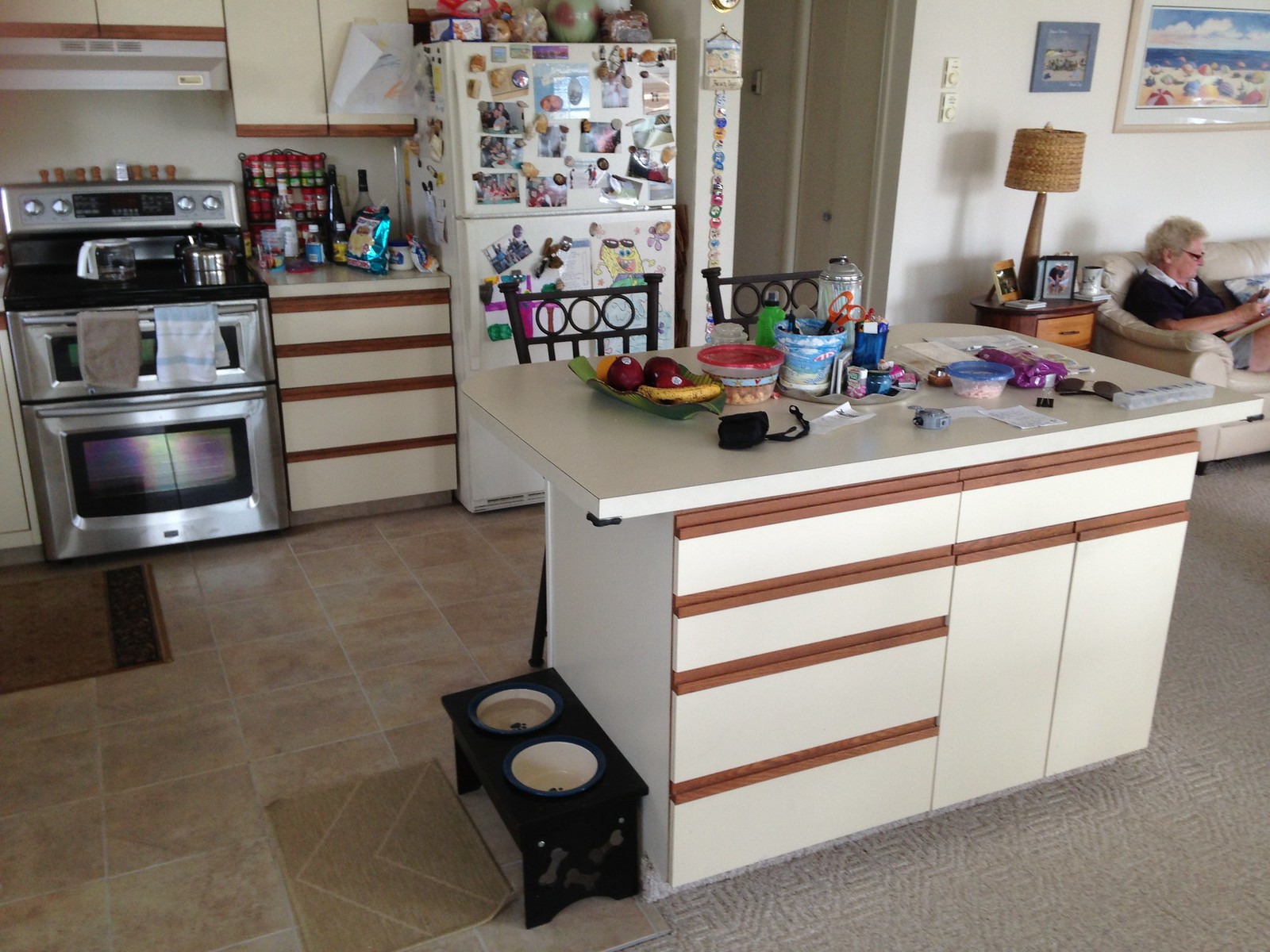This photograph captures an open-concept kitchen and living room, presenting a cozy and lived-in atmosphere. The photo, in landscape orientation, highlights the tidy yet vibrant kitchen on the left and the inviting living room on the right.

The kitchen boasts a brownish beige tiled floor with white grout, creating a subtle yet warm base. A black dog bowl stand with two white bowls, edged in blue, sits in the center against a functional island that bridges the kitchen to the living room. This island, predominantly white with a striking red trim around the drawers, boasts a durable white countertop, seamlessly integrating the two spaces.

In the background, a white refrigerator serves as a focal point, adorned with an array of photos, adding a personal touch. Adjacent to the refrigerator, the cabinetry and drawers, finished in beige with a matching red trim, provide ample storage. The stainless steel stove, complete with an overhead cabinet and smoke hood, hints at a well-equipped cooking area. Several rugs scatter across the kitchen floor, contributing to the room's comfortable vibe.

The living room, to the right, features a neutral palette with a beige solid or spiral-themed floor that complements the beige couch. This cozy seating area, adorned with a lamp and a nightstand, offers a welcoming spot for relaxation. An elderly woman is comfortably seated on the couch, engrossed in reading, adding a sense of homeliness to the scene.